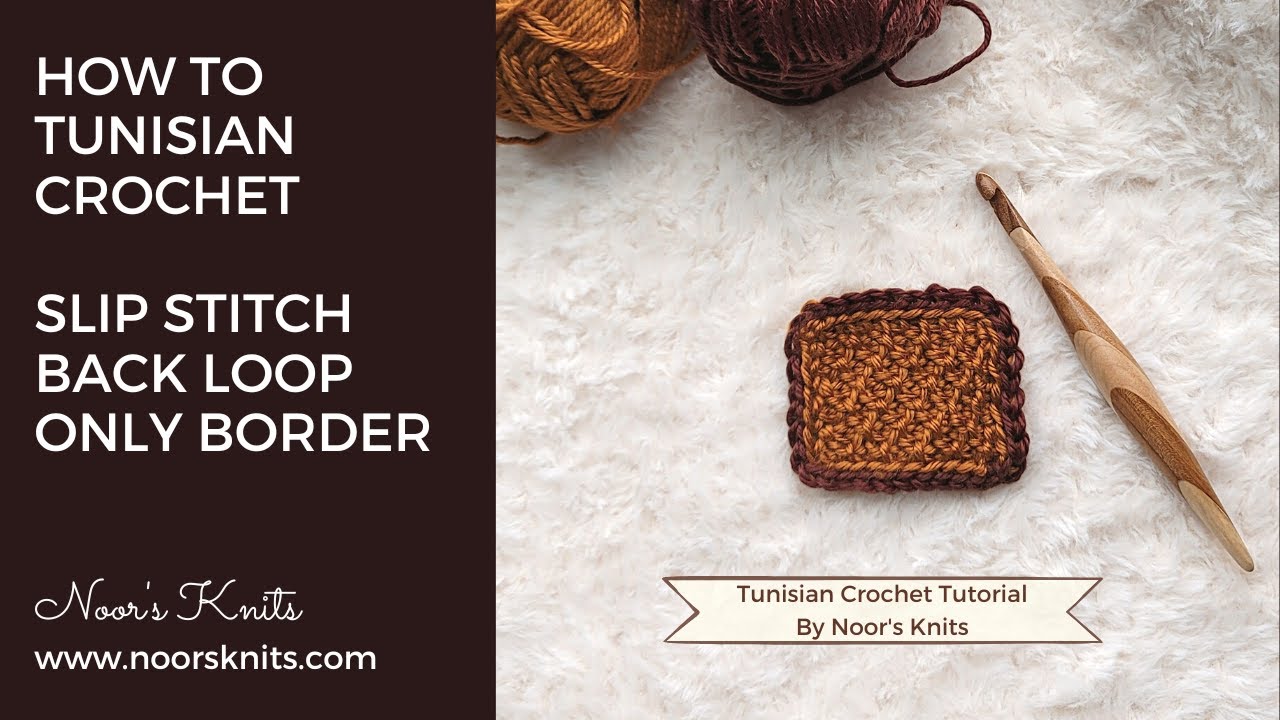This horizontally aligned rectangular digital poster image is divided into two sections. On the left, a vertical dark brown, almost black, rectangle features white all-caps text that reads: "How to Tunisian Crochet Slip Stitch Back Loop Only Border." Below this, in cursive, it says "Knorse Knits," followed by "www.knorseknits.com" in regular text. 

To the right, a square photograph displays an arrangement on a fuzzy white surface, possibly a blanket or rug. Centered in this photo is a small knitted piece, resembling a potholder or coaster, crafted with brown wool and bordered in dark brown. Positioned diagonally to the right of the knitwork is a wooden knitting tool characterized by alternating light and dark brown segments. In addition to the knitting tool, there are two balls of yarn at the top of the photo: the one on the left is light brown, and the one on the right is dark brown. At the bottom of this image part, the text reads: "Tunisian Crochet Tutorial by Knorse Knits."